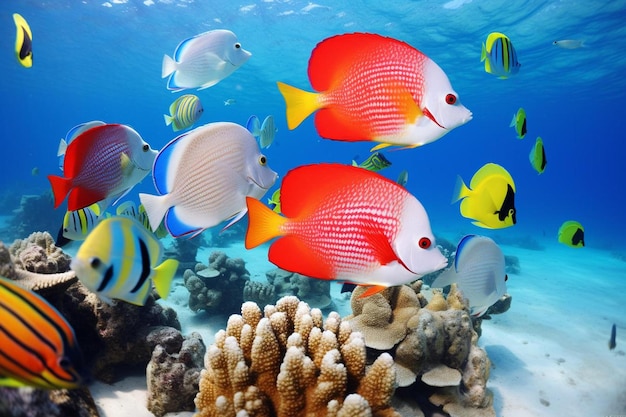This landscape layout photograph captures a stunning underwater scene featuring crystal-clear blue water and a pristine, white sandy ocean floor dotted with various forms of vibrant coral, predominantly in shades of brown and gray. The image is teeming with multicolored fish, creating a lively spectacle. Front and center are two fish adorned in striking shades of red, white, and yellow. To their right swim fish with bold yellow and black patterns, while to their left are predominantly white fish. Off to the side is another fish displaying the same red and white coloration. In the upper left-hand corner, a yellow and white fish can be seen, while the lower left corner showcases an orange and black striped fish accented with yellow. The diverse fish species, including those with combinations of yellow, blue, and black, enhance the mesmerizing beauty of the blue underwater expanse, making it a vivid and dynamic portrayal of marine life. There are no people or text present, allowing the natural underwater environment to take center stage.